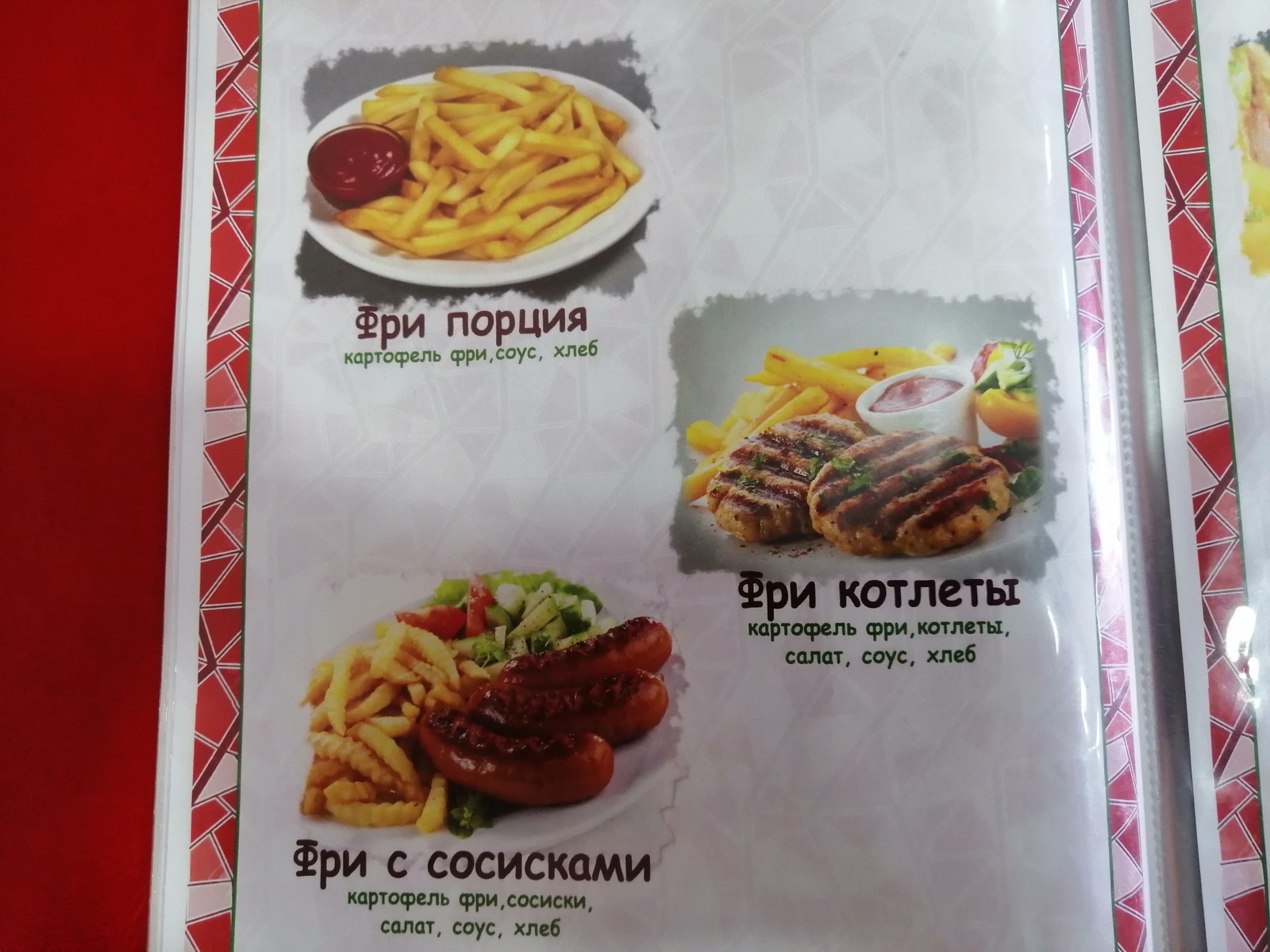This detailed photograph captures a page of a Russian menu laid out on a red table. The visible page showcases three main food options, each labeled with Russian text beneath them. 

At the top left, there is an image of French fries served with ketchup. Moving to the center right, the centerpiece comprises two grilled burgers, marked with distinctive grill lines and garnished with fresh, green herbs. Accompanying the burgers are additional French fries and a dollop of ketchup in a small white cup, along with a backdrop of mixed vegetables. 

At the bottom, the menu features three small sausages, also marked with grill lines, nestled against a serving of crinkle-cut French fries. Adjacent to the fries is a medley of chopped vegetables exhibiting green and red hues. 

To the right edge of the photograph, another page of the menu is partially visible, characterized by red lines and irregular shapes, although its contents are obscured.